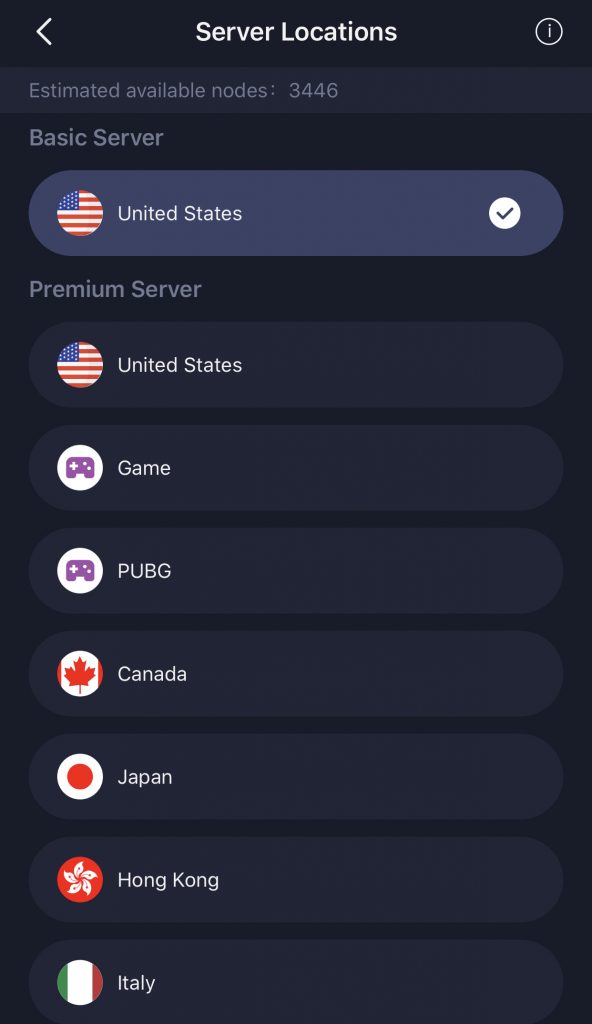The screenshot displays a mobile interface with a dark theme, specifically showcasing various server locations in a VPN app or similar service. The background of the screen is black, enhancing the contrasting elements on the display. At the top of the screen, there is a left-facing triangular bracket, followed by centered white text that reads "Server Locations." On the upper right corner, there's an information icon consisting of a lowercase 'i' enclosed in a white circle.

Below this header is a horizontally aligned section in dark charcoal gray color, displaying the gray text "Estimated Available Nodes: 3446." Next, there is a section labeled "Basic Server" in a larger font size. This section highlights the currently selected server location: the United States. This is indicated by a circular icon featuring the US flag, white text stating "United States" to its right, and a white circle with a gray check mark on the extreme right side of this rounded rectangular box.

Further down, beneath the "Basic Server" section, additional server options categorized as "Premium Servers" are presented. Each option is contained within a similarly styled rounded rectangular box. The available premium server locations and their corresponding icons are:
- United States: represented by a circular icon with the US flag.
- Game: symbolized by a purple game controller icon.
- PUBG: denoted by the same purple game controller icon as the "Game" option.
- Canada: represented by a circular icon with the Canadian flag.
- Japan: indicated by a circular icon featuring the Japanese flag.
- Hong Kong: symbolized by a circular icon with the Hong Kong flag.
- Italy: represented by a circular icon with the Italian flag.